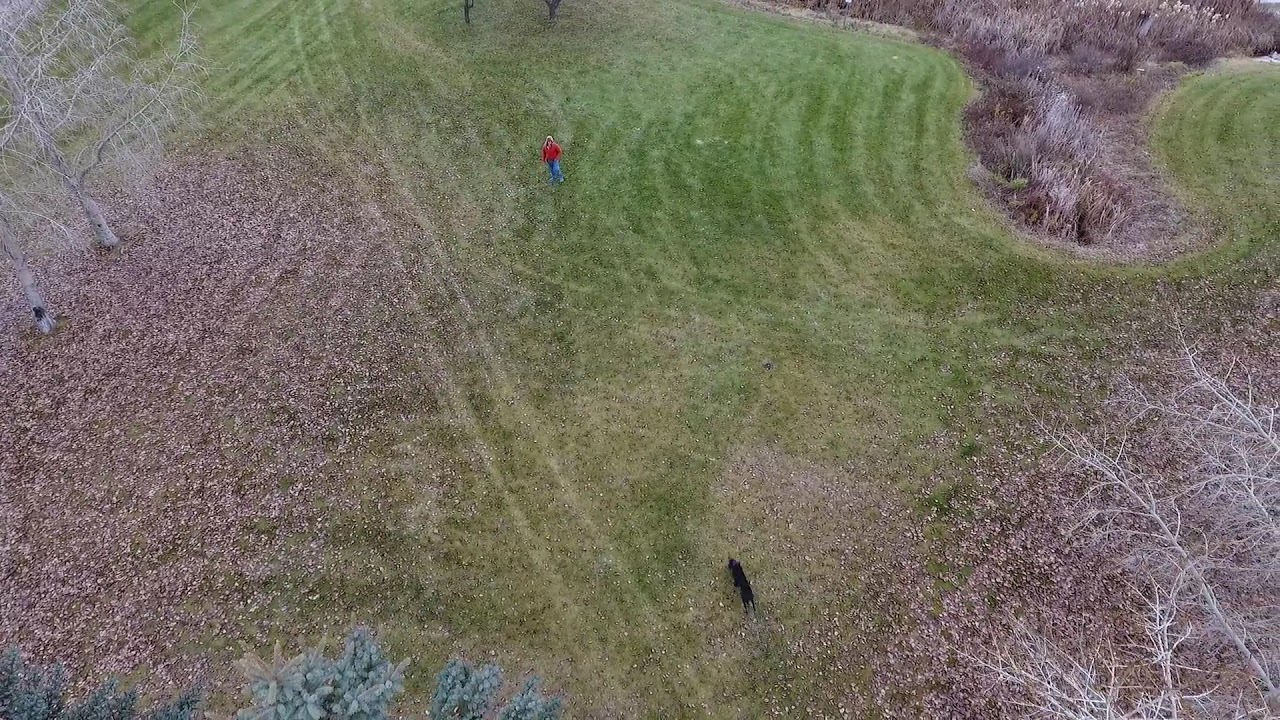The aerial drone shot captures an autumnal scene, looking down on a field characterized by both green grass and scattered brown leaves. On the left side, bare white trees stand, surrounded by piles of fallen leaves at their bases, indicating the end of fall with no snow present. The focal points in this expansive field are a black dog at the bottom center of the image, seemingly stationary and seen from behind, and a woman at the top center of the image. She is wearing a red shirt and blue jeans, holding her arms up, possibly controlling the drone with a device in her hands. The scene suggests it is midday, with ample natural light illuminating the varied hues of brown, green, red, and black. This outdoor setting might be a park, captured in serene stillness as the woman engages with the dog.